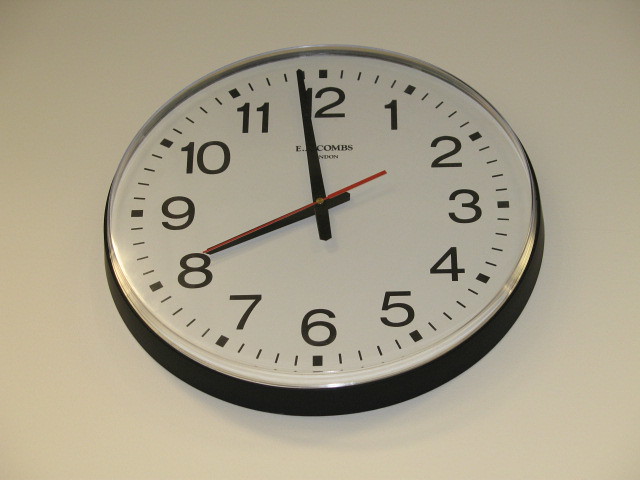This image captures a close-up of a round, professional-looking clock on a smooth, white wall, reminiscent of those typically found in a classroom. The clock features a plain design with a black trim encircling its white face. Bold black numbers mark the hours, each of which is accompanied by a black square box, while individual minute lines are positioned outside these numbers. The clock shows the time as 7:55, with the shorter black hour hand pointing at the 8, and the longer black minute hand nearing the 12. A red second hand adds a touch of color, enhancing readability. Beneath the black hands, part of the name "E. Combs" is visible, although partially obscured by the hour hand. The angle of the photograph, taken slightly from below, places the clock prominently at the center, highlighting its unremarkable yet functional appearance as it methodically displays the time.